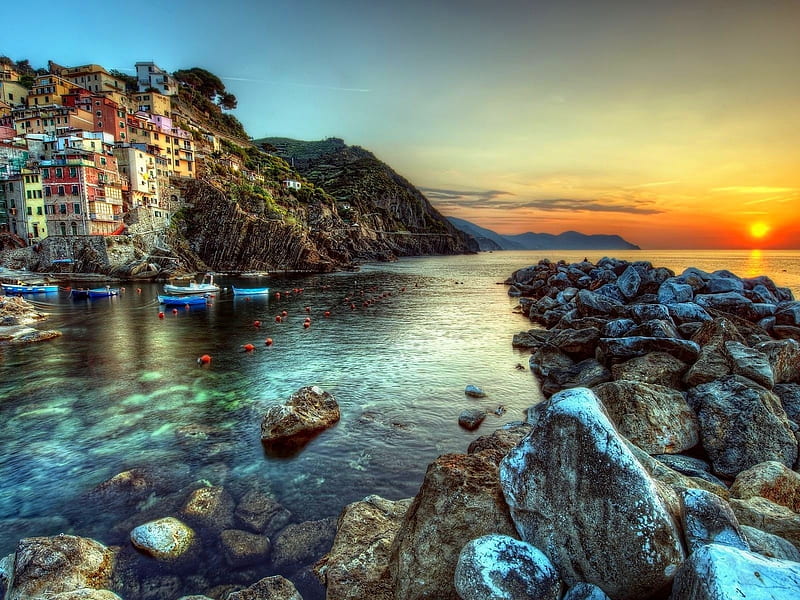This image depicts a picturesque seaside town, reminiscent of the Italian Riviera, with its closely stacked buildings cascading down a steep hillside towards the water. The scene is captured from the perspective of someone standing on a rock formation that serves as a wave barrier near the shore. In the foreground, shallow rocky waters reflect various hues of blue and dark colors, while small blue boats and buoys float nearby. To the left, houses painted in vibrant shades of yellow and pink dot the hillside, creating a charming, densely-built townscape. Out on the horizon, majestic mountains rise, framing the setting sun that casts a golden glow across the lower sky and water, contrasting with the blue sky that dominates the upper part of the image.